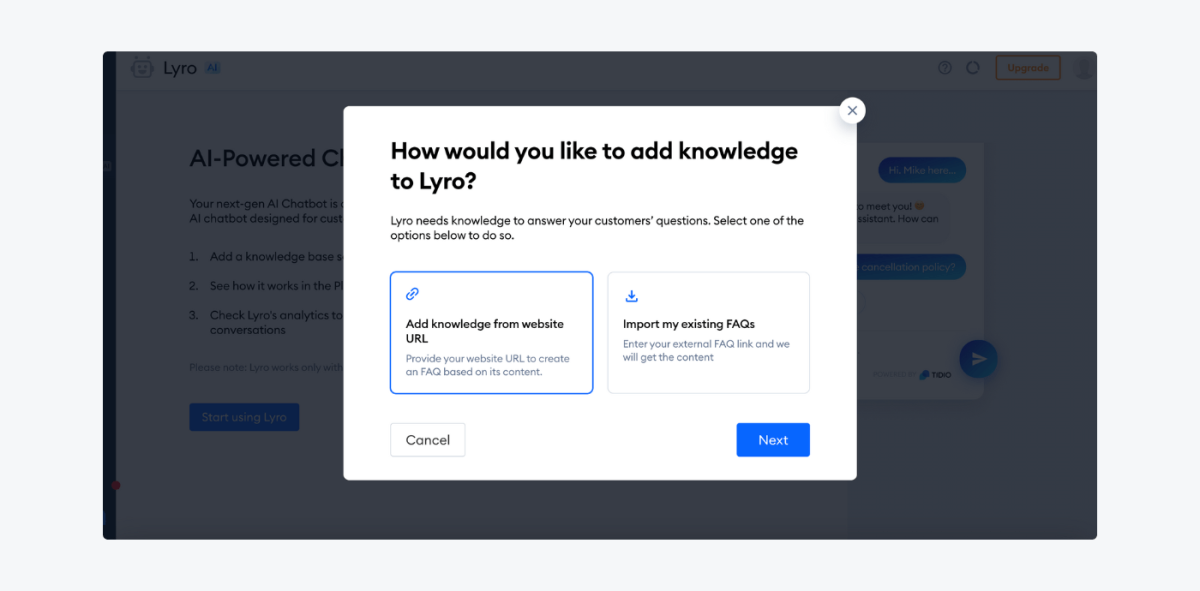The image appears to be a screenshot from a website featuring a semi-transparent, grayed-out background with a large, white pop-up window overlay. In the background, a white banner at the top bears the word "Lira" or "Liro." Below the banner, although partially obscured and grayed out, is text that reads "AI-powered..." followed by a cut-off section, and a short sentence that ends with an ellipsis.

To the right of this text, additional content is visible but difficult to read due to its small size and faded appearance. It includes numbered items such as "1. Knowledge Base" and "2. See How It Works," with a partially readable "3. Check Lira's Analytics..." among other text elements that remain unreadable.

The focus of the image is the white pop-up window which asks, "How would you like to add knowledge to Liro?" Below this question are two options presented in rectangular boxes: "Add knowledge from website URL" and "Import my existing FAQs." At the bottom right of the pop-up window is a blue button with white lettering that reads "Next."